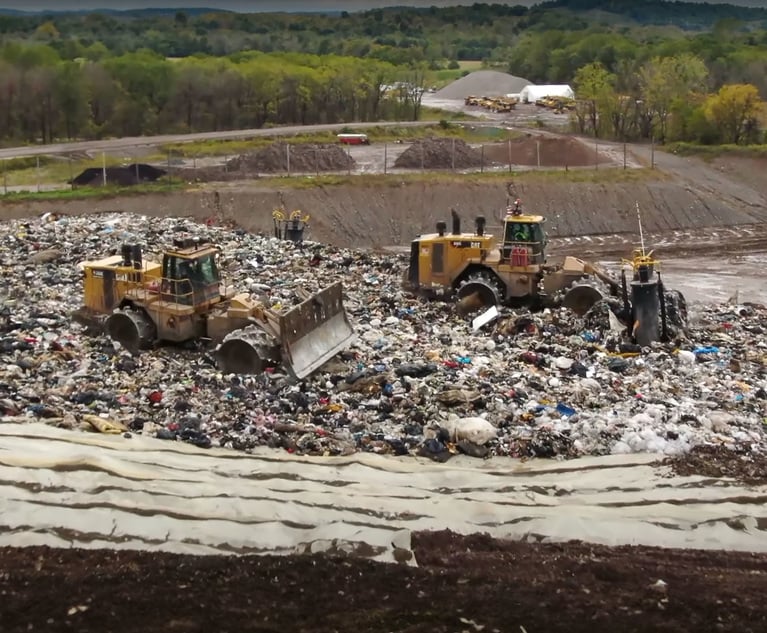This detailed photograph is a square image capturing a bustling construction scene. In the foreground, there are two large yellow earth-moving machines, possibly backhoe loaders or bulldozers, distinguished by their substantial metal scoops and pusher devices. They sit amidst a significant pile of rubble and debris, suggesting activity that might involve either demolition or clearing of trash. Surrounding them is a mixture of bare dirt and strips of material—possibly paper—strewn along the ground, adding to the disordered state of the site.

Further back, the image transitions into an empty, barren field that stretches towards the horizon. Beyond the field, a house is visible, standing before a dense wooded area filled with green trees. A road snakes off into the distance, hinting that the construction work might be intended for road development or some other structure-building project. Additionally, a parking lot can be seen with more construction vehicles lined up and a large gray gravel pile.

To the right in the background, there's a noticeable chain-link fence atop a slope, with water running next to it, providing a clear boundary between the construction site and the more natural landscape of dense trees beyond. This detailed scene paints a vivid picture of an active, possibly transformative, construction effort under a vast, open sky.